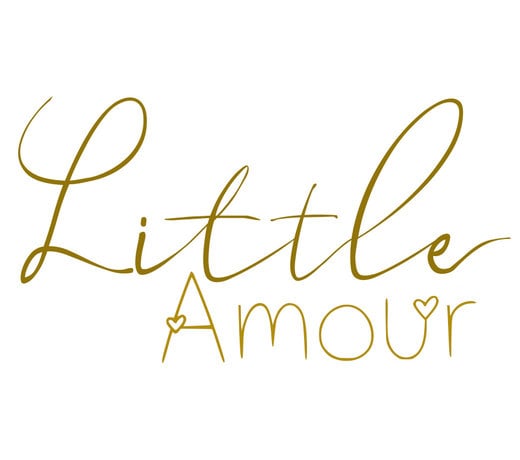The image features a white background with elegant gold text. At the top, the word "little" is written in an elaborate cursive style, much larger and more intricate, with notable details such as a traditional looped cursive 'L' and a small loop on the first 'T'. The word "amour" is positioned below "little", aligned so that "amour" begins where "little" ends. "Amour" is rendered in a lighter gold, non-cursive, hand-printed font. Unique decorative elements include a small heart where the horizontal crossbar of the capital 'A' intersects with its left stroke and another heart at the end of the 'U'. Overall, the typography blends the flowing elegance of cursive with the charming simplicity of print, enhanced by subtle heart details.